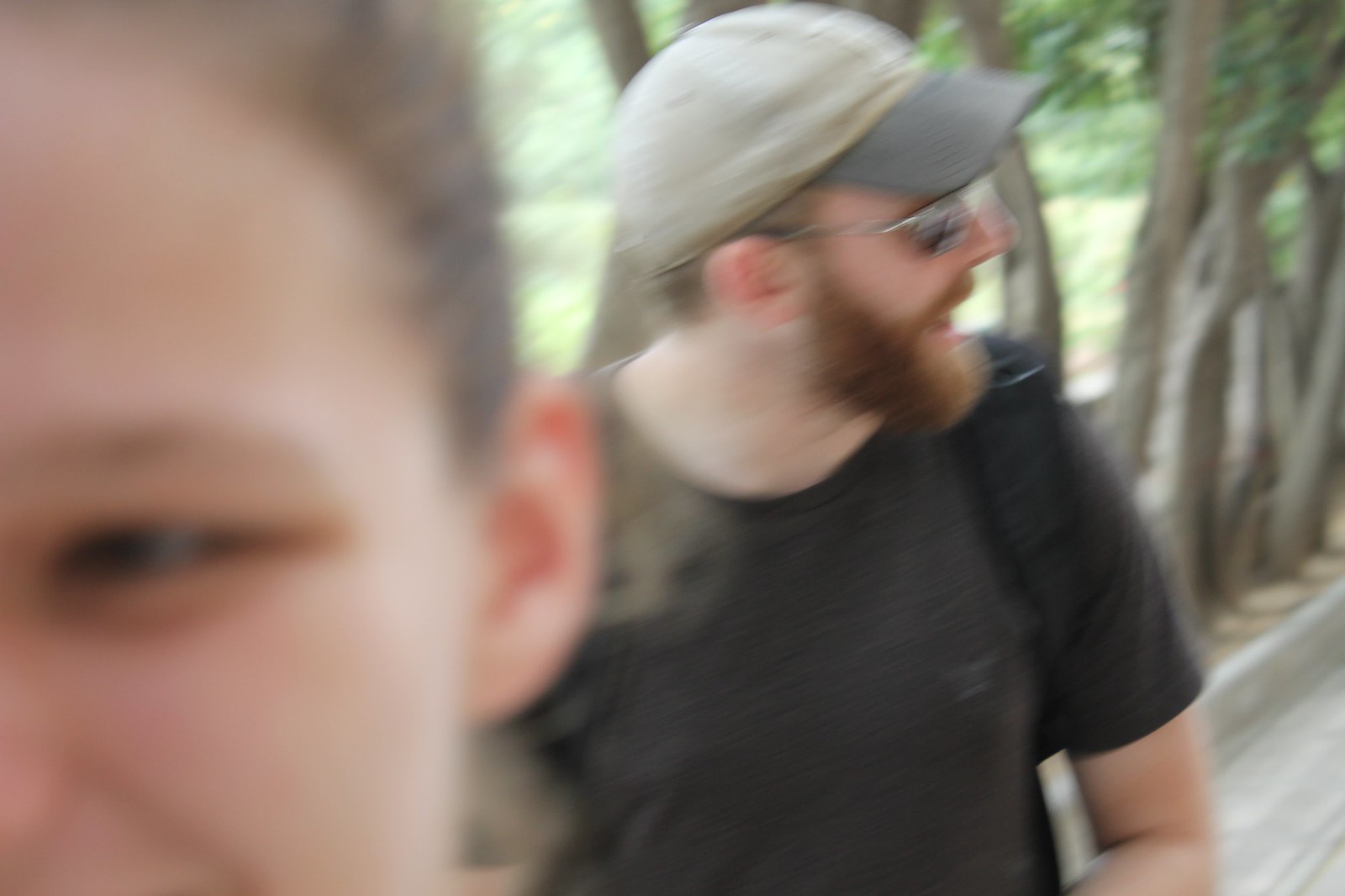In this blurry, out-of-focus image, taken in motion, we see two people outdoors on a concrete walkway lined with slender trees with brown trunks and green leaves against a backdrop of a grassy field. On the left, there is a very up-close and indistinct portion of a face, showing an eye, an ear, and some hair, possibly that of a girl with short brown hair tied back in a ponytail. The primary focus, however, seems to be on the person slightly behind her. This individual is a white man wearing a black short-sleeved shirt, a light gray or khaki-colored baseball cap with a darker brim, aviator-style sunglasses, and possibly black backpack straps. He has a noticeable ginger beard and mustache and is turning his head to the side, while his body faces forward. The overall composition suggests an impromptu photo capturing a moment of casual movement in a serene, leafy outdoor setting.